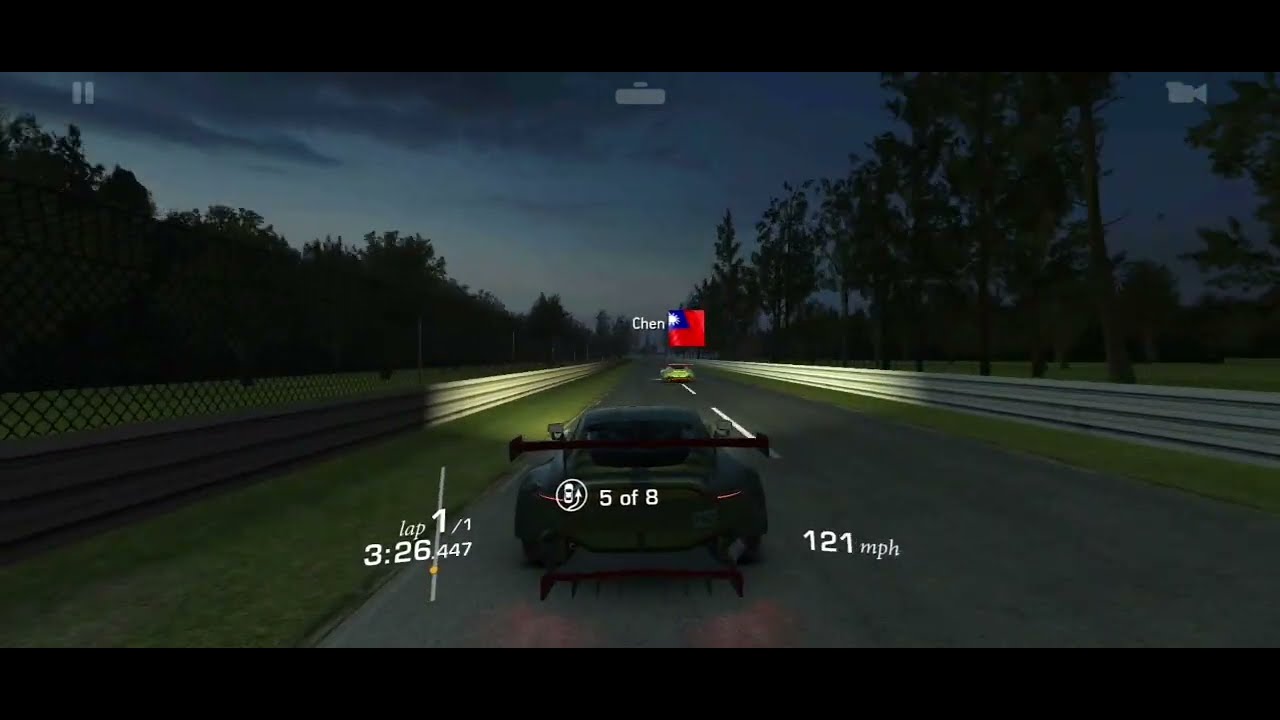This is a detailed screenshot from a racing video game set during dusk with a light bluish sky turning dark, filled with dark clouds. The road in the middle features two cars: a gray Porsche with a prominent tail fin trailing behind a yellow car. The gray Porsche has a text overlay above it reading "5 of 8" in white, and additional texts to the left and right of it display "lap 1/1 3:26.447" and "121 mph," respectively. A Singapore flag and the name "CHEN" are displayed above the yellow car in front. Both sides of the road are bordered by strips of grassland, metallic boundary fences, and tree-lined peripheries, enhancing the scene's realism. A camera icon is also visible in the top right corner of the screen, adding to the game's immersive interface.